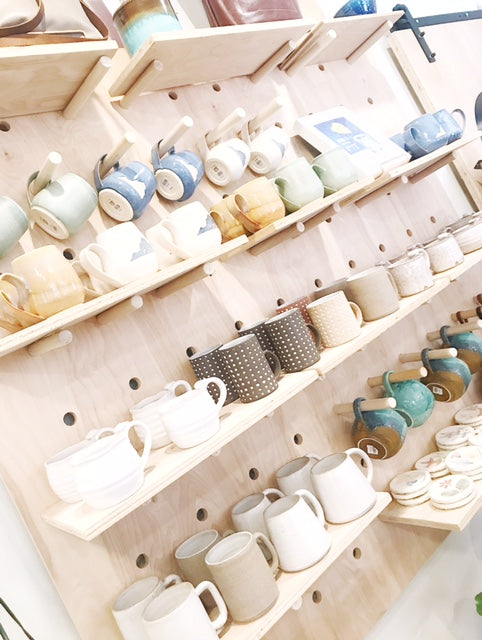This image features a vertical, rectangular display on a white wall, showcasing a collection of large, beautifully designed coffee cups. Central to the display is a light-colored wooden cupboard system with adjustable shelves formed by horizontal light brown wood planks. The top shelf's contents aren't visible, but below it, five wooden pegs hold coffee cups in hues of beige, pale green, and pale blue. The remaining three visible shelves are adorned with an array of colorful coffee cups, including shades of blue, beige, and pale green. The second shelf features beige cups alongside brown cups adorned with white polka dots. Cups hanging from pegs below exhibit a striking teal color with brown bottoms. The bottom right section of the image shows additional coasters and more peg holes for flexible cup arrangement, highlighting the cupboard's functional yet aesthetic design.